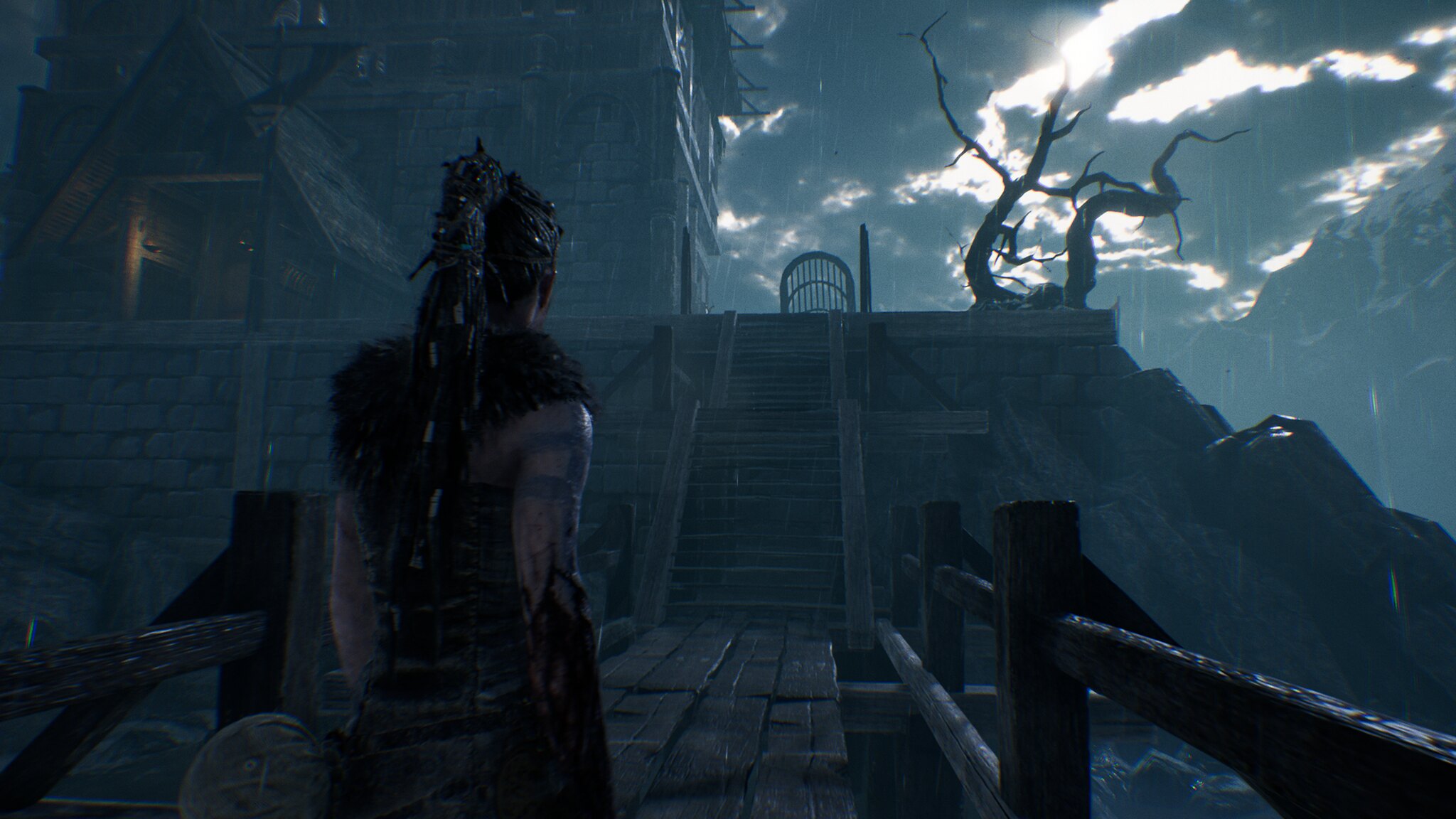In this screen capture from a video game, we are presented with an atmospheric night scene. The main focus is the back of a character standing at the base of a staircase that ascends to a building or home. The character is donned in a fuzzy vest or stole and sports long hair intricately braided into a mohawk that cascades down their back. The setting is drenched in rain, enhancing the dark and ominous mood. On the right side of the image, a wooden fence railing is partially visible, while to the left, we can see the edge of the building. The overcast sky is heavy with clouds, contributing further to the gloomy ambiance. Completing the scene on the right side is a stark, leafless tree, its branches appearing ragged and forlorn against the stormy backdrop.